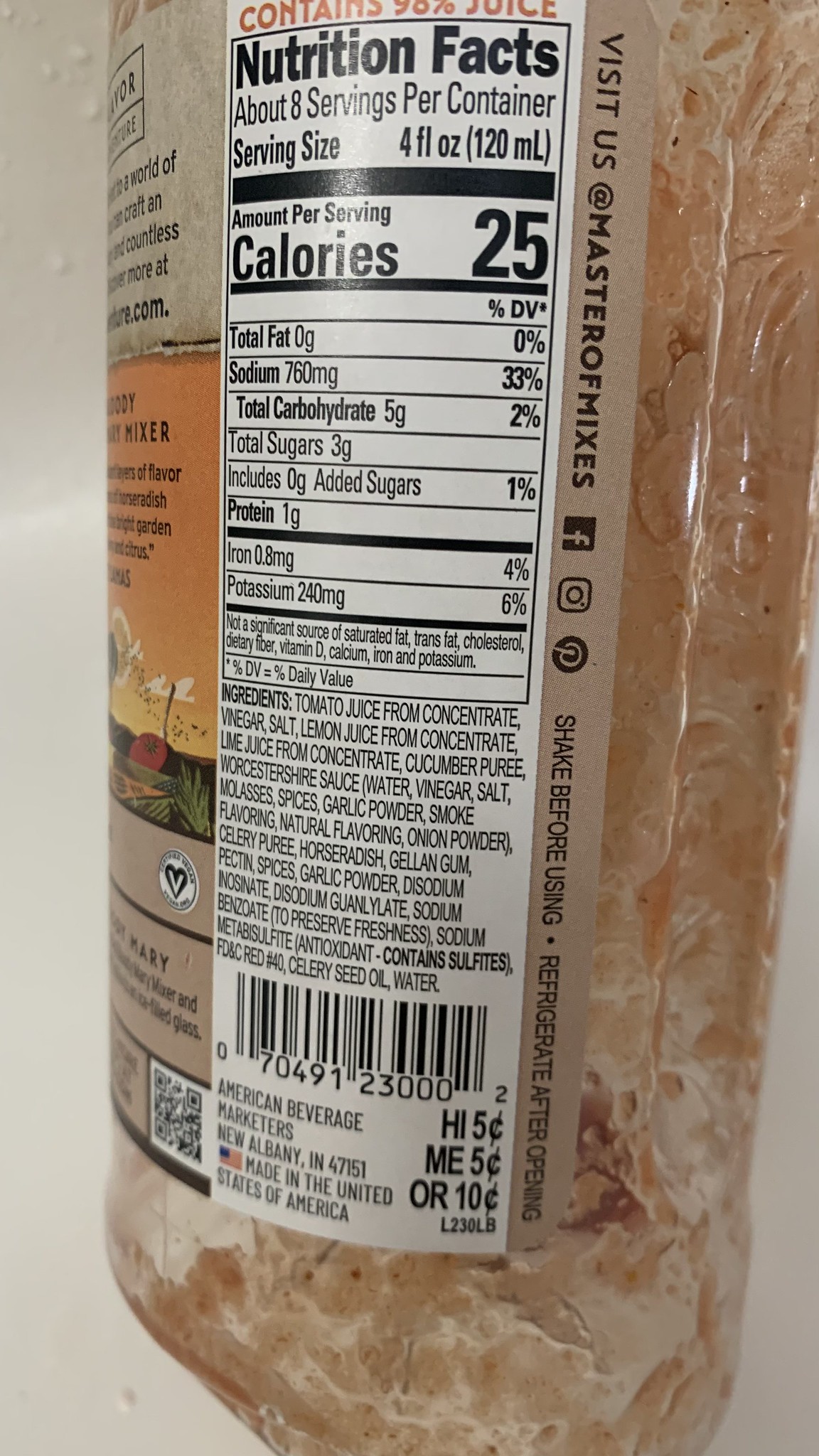The image showcases the back label of a mostly empty bottle of a juice product, likely a vegetable-based beverage given its ingredients. The bottle is predominantly beige with natural, rocky marble-like orange patterns. The nutrition label, front and center in the image, details that it contains 98% juice and only 25 calories per serving, with eight servings per container. Key ingredients include tomato juice from concentrate, vinegar, salt, and lemon and lime juices from concentrate. Other notable features on the label include a QR code, a reference to social media logos for Facebook, Instagram, and Pinterest, and the instructions to shake well before using and refrigerate after opening. It mentions the manufacturer's name—American Beverage Marketers—along with an address in Indiana, and recycling information for various states. The bottle's design and color give it an opaque appearance, obscuring its contents.